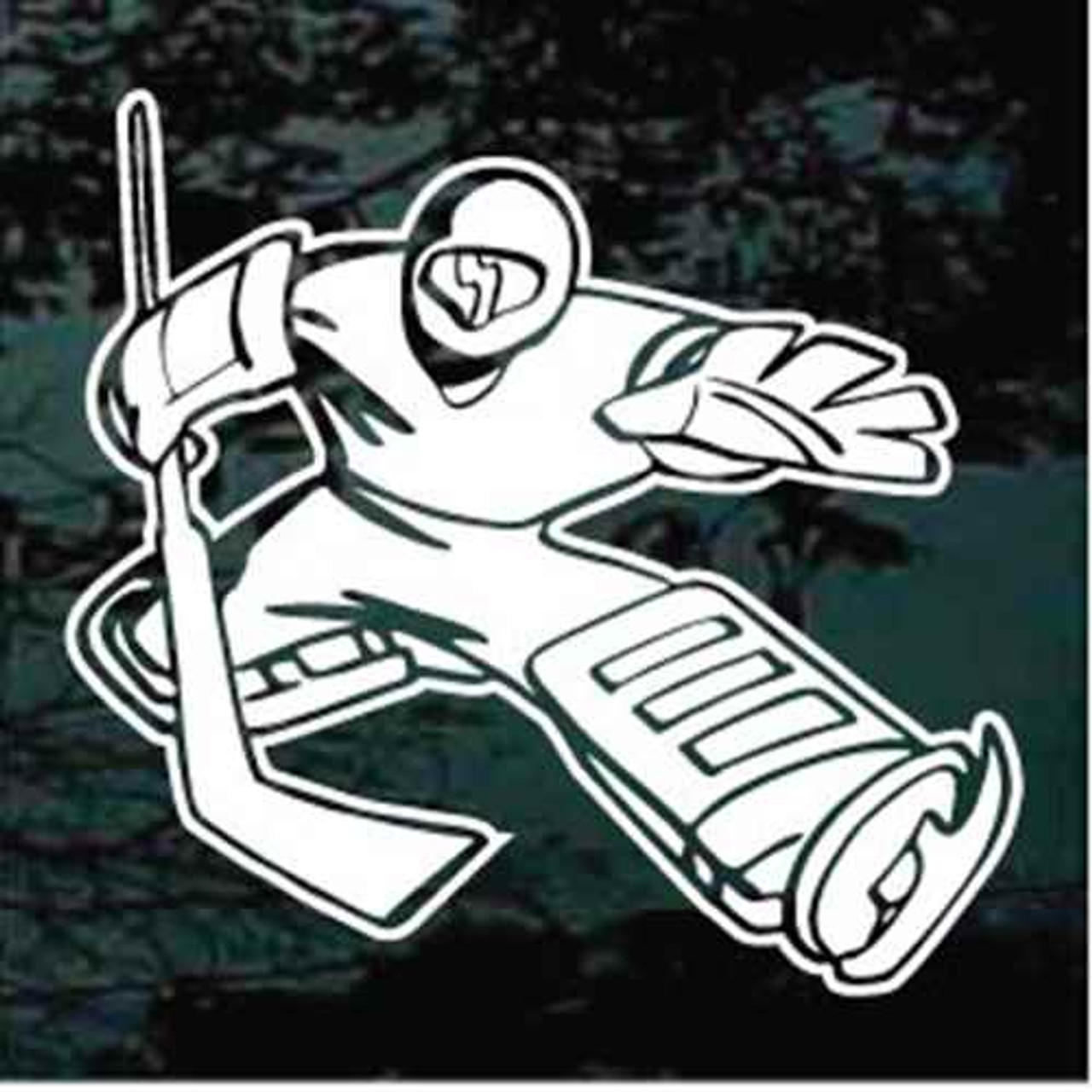The image depicts a stylized, cartoon-like drawing or decal of a hockey goalie in an action pose, possibly blocking a shot. The goalie is predominantly white, accented with black or gray artistic outlines and shading. Dressed in full protective gear, the player wears a white shirt, white pants, shin guards with three downward diagonal slots, large gloves, skates, and a helmet with an obscured face, although the nose is visible. The right arm holds a hockey stick, and one hand is extended outward. The entire illustration is set against a green, tree-like backdrop with black and darker teal branch shapes, giving the impression of an underside view of trees. The image has a balanced, square form, approximately 8 by 8 inches, and does not include any text or real-life photos.